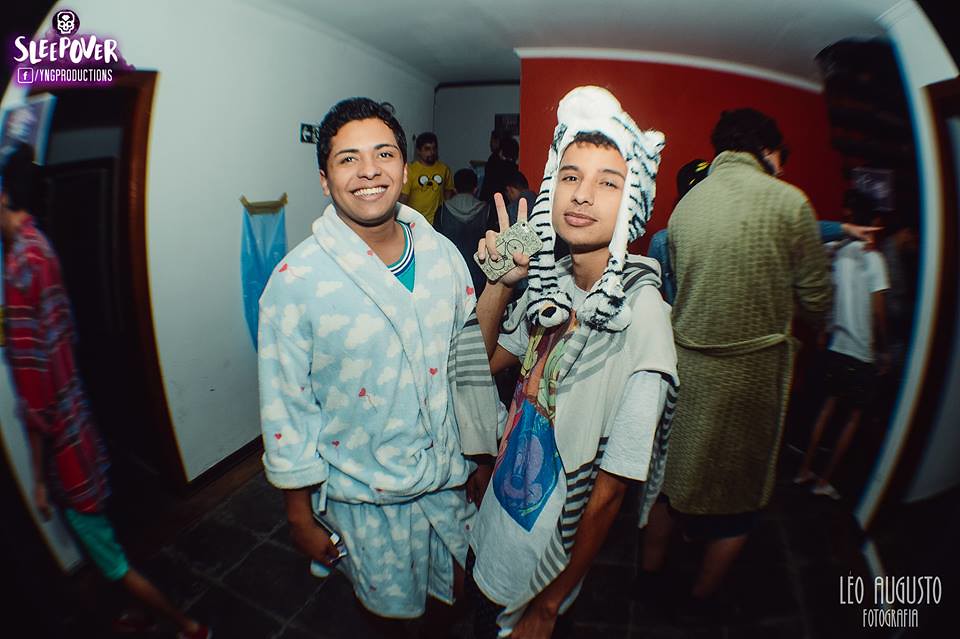In the center of this horizontally-oriented, fisheye-distorted image, there are two young men with medium-dark skin posing for the camera at what appears to be a sleepover party. The man on the left is smiling broadly and wearing a fuzzy, cloud-like robe that is fastened over a blue shirt with white trim around the collar. The man on the right, holding up a peace sign with his right hand and a phone in his left hand, is dressed in a quirky ensemble: striped pajama pants, a really long t-shirt, and a zebra-striped hat with paw-like extensions that hang down around his face, along with a striped sweater draped over his shoulders.

The background features a red wall and a white wall off to the side, along with other people in robes and t-shirts, reflecting the sleepover theme. In the upper left-hand corner of the image, there is white text that reads "Sleepover" along with a logo for "YNG Productions" and a Facebook symbol, all set against a purple haze. The credit "Leo Augusto Fotografia" is displayed in the bottom right-hand corner.